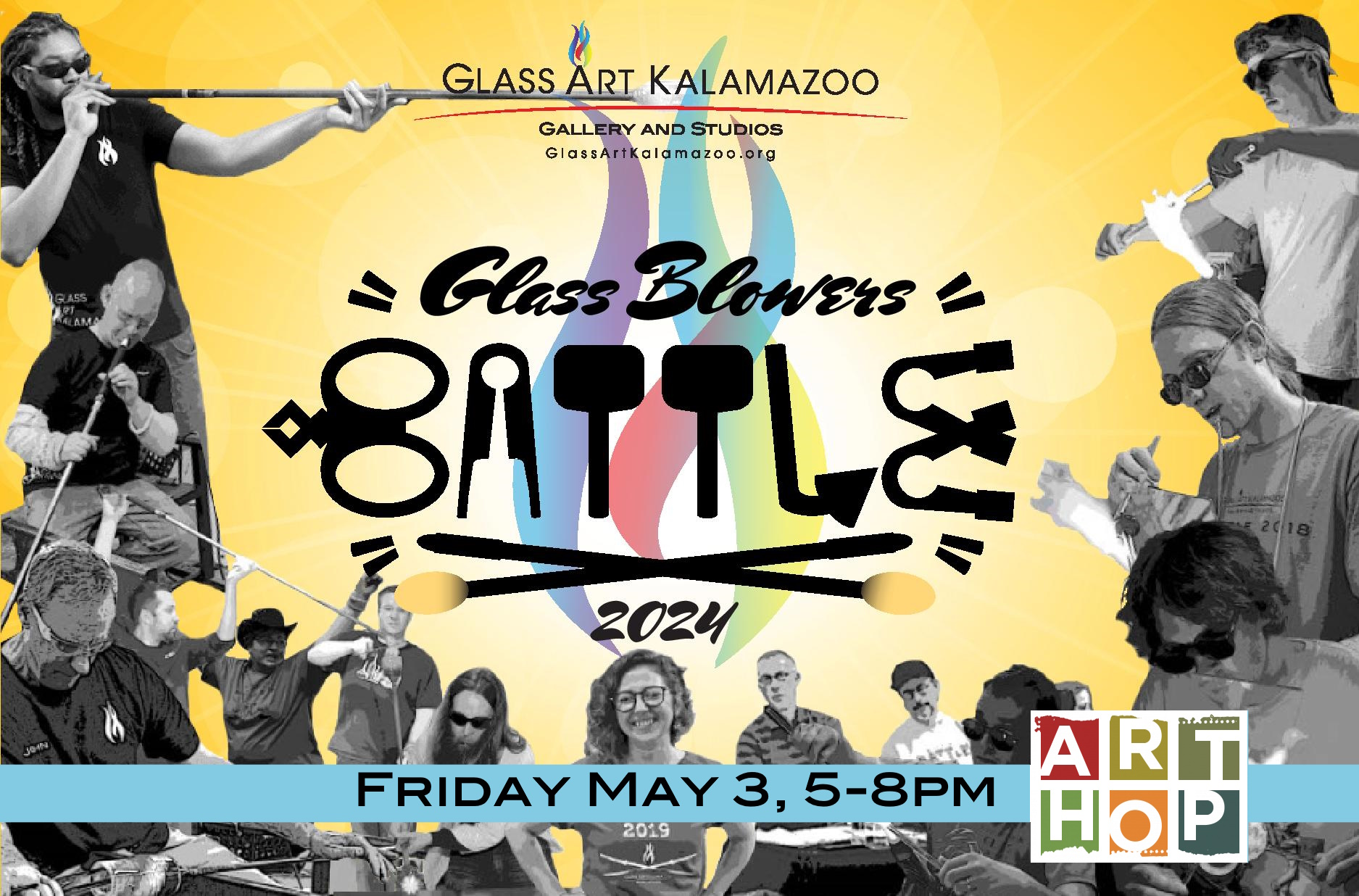This vibrant advertisement for the Glass Blowers Battle 2024 is set against a yellow background with varying shades. Dominating the top of the image, bold text proclaims "Glass Art Kalamazoo," followed by "Gallery and Studios, GlassArtKalamazoo.org." Centrally located, large black bold letters announce "Glass Blowers Battle 2024." Beneath this, more text details the event's date and time: "Friday, May 3rd, 5 to 8 p.m.," alongside the phrase "Art Hop."

At the heart of the design is a multicolored flame motif featuring hues of red, yellow, greenish-yellow, blue, and purple. This dynamic centerpiece is flanked by black-and-white images of people engaged in the art of glassblowing. These portraits, appearing both on the left and right sides of the flame and extending towards the bottom of the image, capture the artisans in various poses. The bottom of the advert is filled with more of these monochromatic images, melding the artistic flair of the flame with the craftsmanship of the glassblowers. The composition is crafted to convey the excitement and creativity of the upcoming event in Kalamazoo, Michigan.